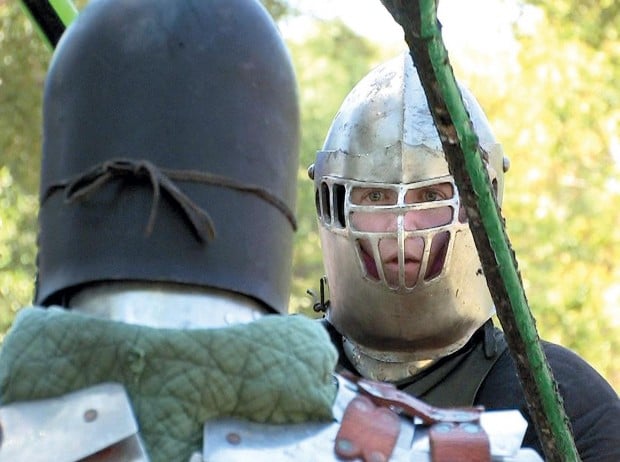This daytime outdoor photo captures a scene that appears to be from a medieval reenactment. The background reveals a forest with blurred trees and greenery on both sides. In the foreground, there are two individuals dressed in homemade medieval armor. The person on the right wears a shiny silver metal helmet with holes for visibility, exposing some facial features such as eyes, nose, and mouth. Dressed in black armor, he holds a long green staff or spear. The individual on the left, partially turned away from the camera, sports a black helmet secured with a brown leather strap and wears padding with green around the neck. Their armor, similarly handmade with elements of leather, suggests the authenticity of their role-playing attire. Both appear to be engaged in an activity, possibly involving the green and black spears they each hold.